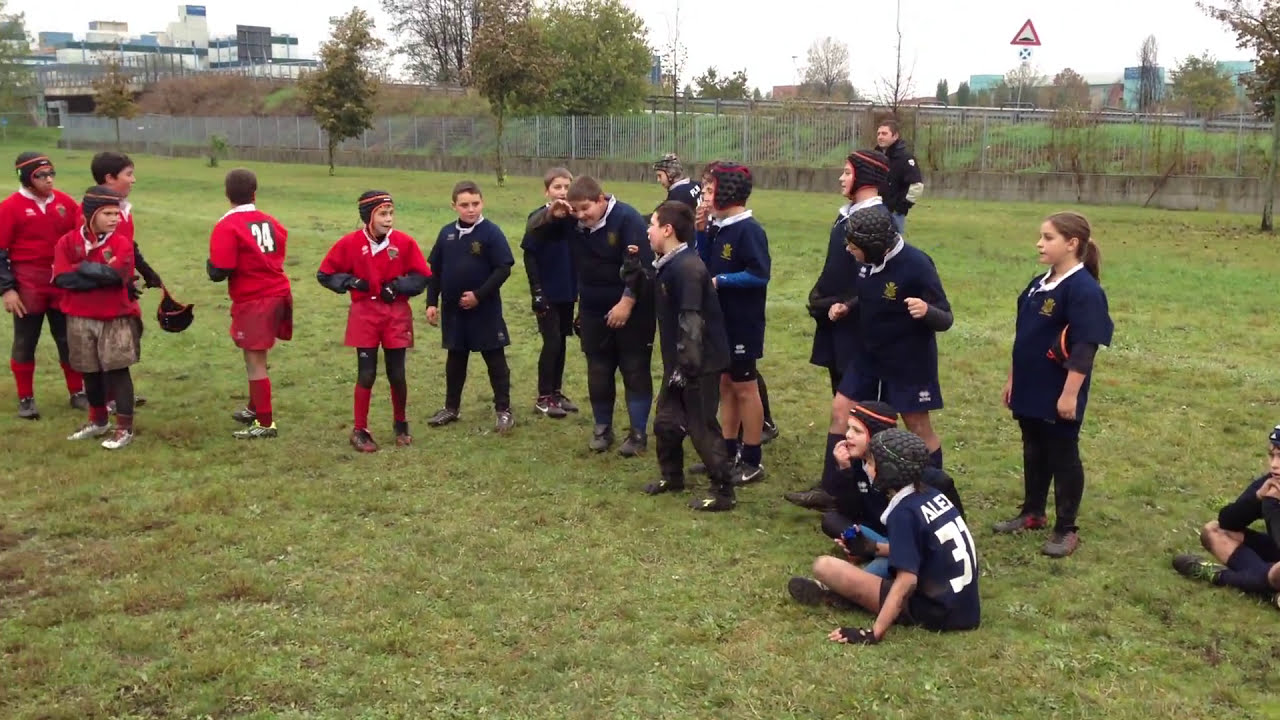The photograph captures a vibrant scene in a park on an autumn day, with two teams of middle school children, aged around nine or ten, poised for a game on a large grassy field. The field is surrounded by a mesh metallic fence and framed by tall, leafy green trees. The sky above is a hazy white suggesting it's midday. The children are divided into two distinct teams; one team is dressed in dark navy blue (appearing almost black), while the other team is bedecked in bright red uniforms, complete with matching T-shirts, shorts, and socks. Some children are wearing knit hats with earflaps, indicating the chilly weather.

Central to the image is a confrontation between a child from the blue team and a child from the red team. They face each other tensely, with a young boy positioned between them, possibly mediating the argument or exacerbating it. Scattered around them, a couple of children sit on the ground observing, while others stand by, watching the scene unfold. In the background, an adult wearing a long-sleeved jacket and jeans approaches the group, perhaps to intervene or supervise. Further behind, the hints of commercial buildings peek through the trees, grounding the scene in a suburban setting.